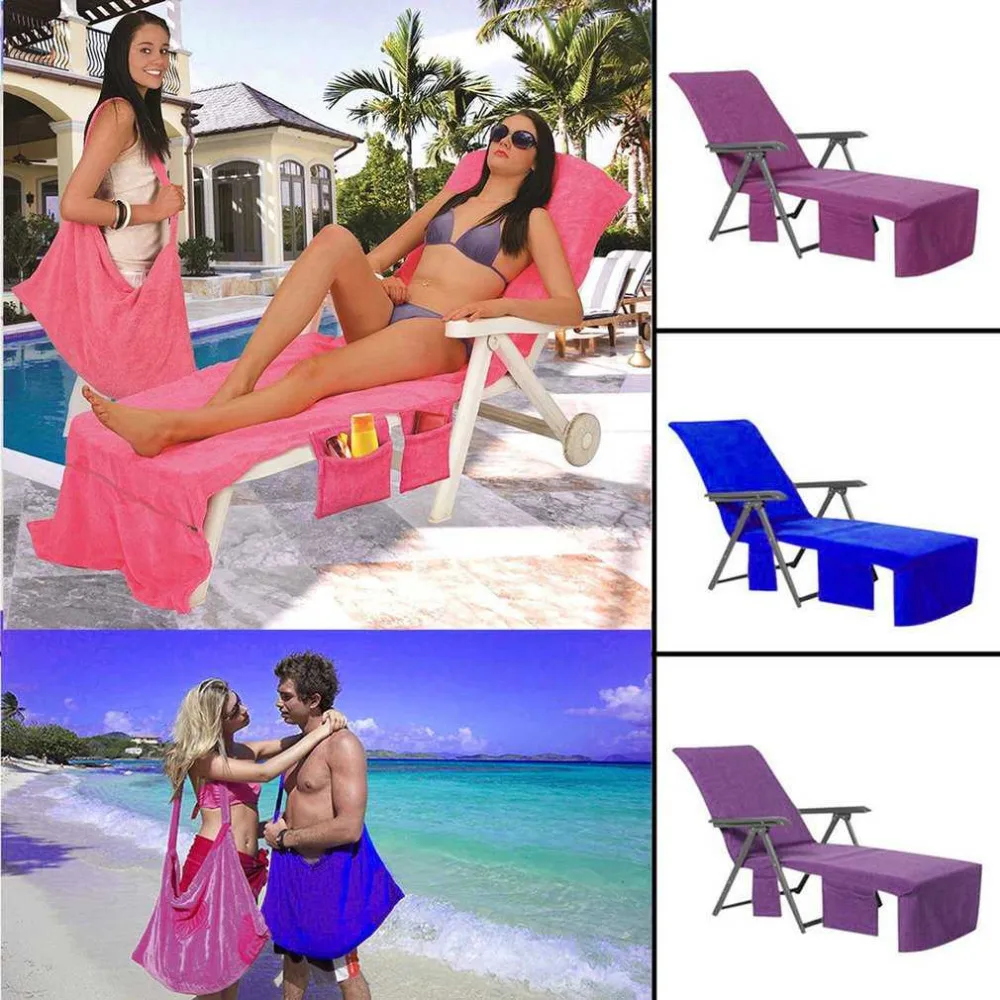This composite image appears to be an advertisement for a microfiber beach lounge chair cover, showcasing its versatility and various color options such as pink, gray, blue, and purple. The main image is divided into five smaller photos, each depicting different aspects of the product in use and set predominantly in a tropical, outdoor environment, likely near a beach.

In the top left photo, two women are at a poolside; one is relaxing on a lounge chair fitted with the cover while the other is carrying the cover in the form of a tote over her shoulder. Visible in the background is a house, adding a residential touch to the scene. At the bottom of the image, a man and a woman are seen enjoying a day at the beach, each carrying the chair cover folded neatly into a tote.

To the right, there are three individual images showcasing the beach lounge chair covers in different colors. The design includes convenient storage pockets on the sides, demonstrating the product's practicality. The entire composition captures the cover's full length, running from the headrest down to the feet, and its ability to be easily carried as a tote, highlighting both its functionality and its aesthetic appeal.